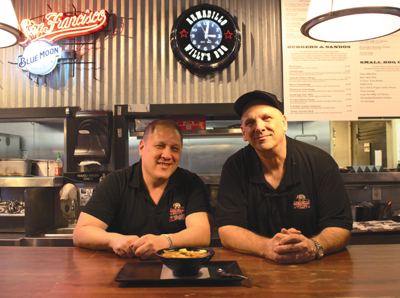The image captures the vibrant interior of a lively eatery, likely a diner or restaurant. Central to the photo are two chefs, one Caucasian and one Asian, who stand behind a welcoming wooden counter, leaning slightly towards each other with warm, friendly smiles. Both chefs are dressed in identical black polo shirts adorned with a brand logo, though the details of the logo remain unclear. The chef on the right complements his uniform with a hat.

In front of them on the counter sits a tray holding a black bowl filled with food, accompanied by a spoon, hinting at the establishment's culinary offerings. The background is rich with visual details: a prominent menu is displayed on the wall, though its specifics are too distant to discern clearly. Above the chefs, a neon sign with "San Francisco" glows in a vibrant orange hue, alongside another neon sign featuring the Blue Moon logo. Adding to the decor, a clock with a black border and the inscription "Armadillo Willie's Barbecue Baby" ticks nearby, enhancing the cozy, eclectic atmosphere of the restaurant.